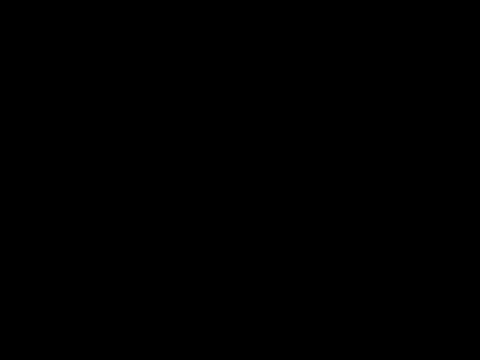The image depicts a uniformly black rectangle stretching across the frame in a landscape orientation, appearing longer than it is tall. The rectangle is solid black with no gradations or variations in shade, maintaining a consistent color throughout. The black is not the deepest hue but rather an extremely dark gray. The image contains no text, objects, or people, and the consistent blackness extends uniformly across the entire frame, giving the impression of a blank TV screen turned off or a canvas entirely painted black.